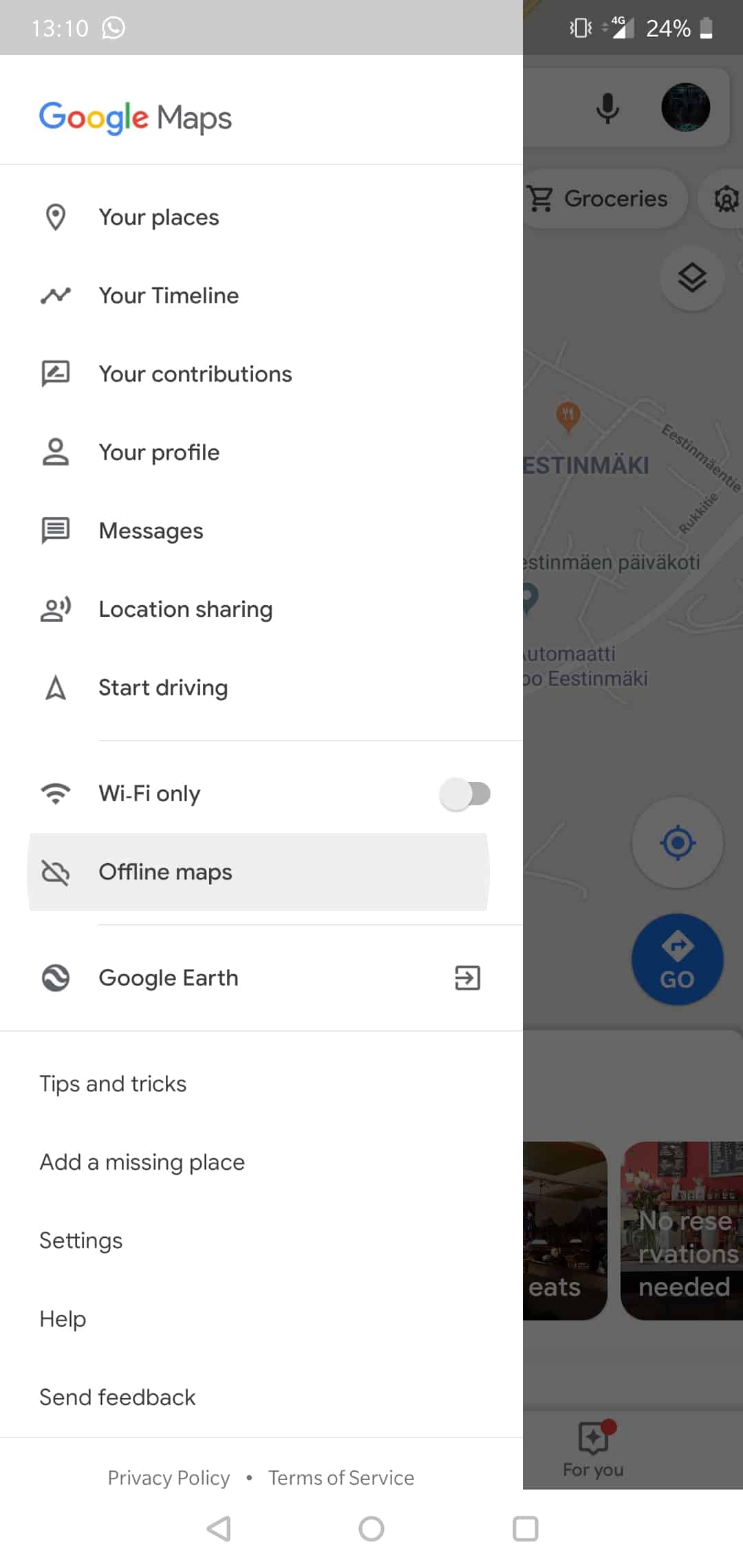This image depicts a smartphone screen interface displaying a navigating app, most likely Google Maps. On the left-hand side, there is an index of options, including 'Your places' marked by an icon, 'Your timeline' represented by a zigzag line, 'Your contributions' illustrated by a speech bubble with lines, 'Your profile' indicated by a person icon, 'Messages' denoted by a speech bubble with lines, 'Location sharing' represented by a person with radiating lines, and 'Start driving' highlighted with an upward-pointing triangle.

On the right-hand side, a section is grayed out, showcasing a partial map view overlaid with an icon labeled "groceries." At the top of this section, there is a speech bubble containing a phone icon, followed by a horizontal line, a vertical rectangle, another line, and an icon representing a right-angle triangle labeled "4G." The status bar indicates '24%' next to a gray battery icon showing that the battery is 24% charged. Above this section, the time displayed is '13:10.'

The main view includes a blue button with a diamond shape and a right-pointing arrow labeled "Go." Towards the bottom, there are a few thumbnail images.

Stretching across the entire top of the screen, there is the Google Maps logo featuring "Google" in its signature colors: blue 'G', red 'o', yellow 'o', blue 'g', green 'l', and red 'e', followed by the word "maps."